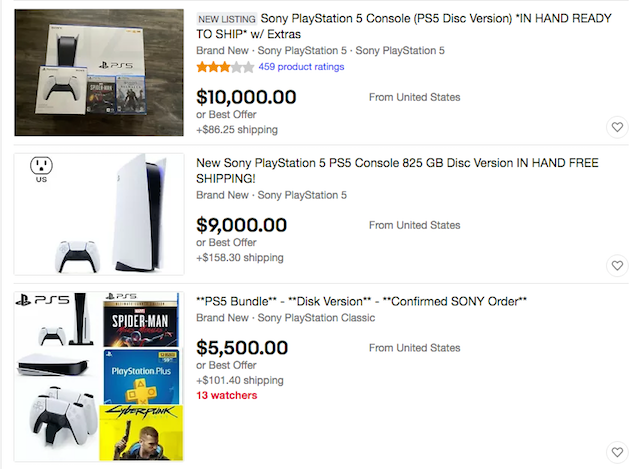The image features a webpage contrasting three different Sony PlayStation 5 listings on eBay, all displayed against a stark white background. On the left side, there are three vertically stacked images of the PlayStation 5 console. Each image is accompanied by a product description box to its right. 

At the top, the description reads: "New listing: Sony PlayStation 5 console (PS5) Disc Version with Extra Accessories. Condition: Brand New. Rating: 3 out of 5 stars based on 459 product ratings. Price: $10,000 or Best Offer. Shipping: $86.25 from the United States."

The middle description advertises: "New Sony PlayStation 5 (PS5) Console, 825GB Disc Version. Availability: In Hand with Free Shipping. Condition: Brand New. Price: $9,000 or Best Offer. Shipping: $158.30 from the United States."

The bottom listing promotes: "PS5 Bundle Disc Version. Confirmed Sony Order. Condition: Brand New. Price: $5,500 or Best Offer."

This detailed view emphasizes the high prices and varying shipping costs for the highly sought-after PlayStation 5 consoles, with options ranging from individual units to bundles, reflecting the competitive and fluctuating market on eBay.